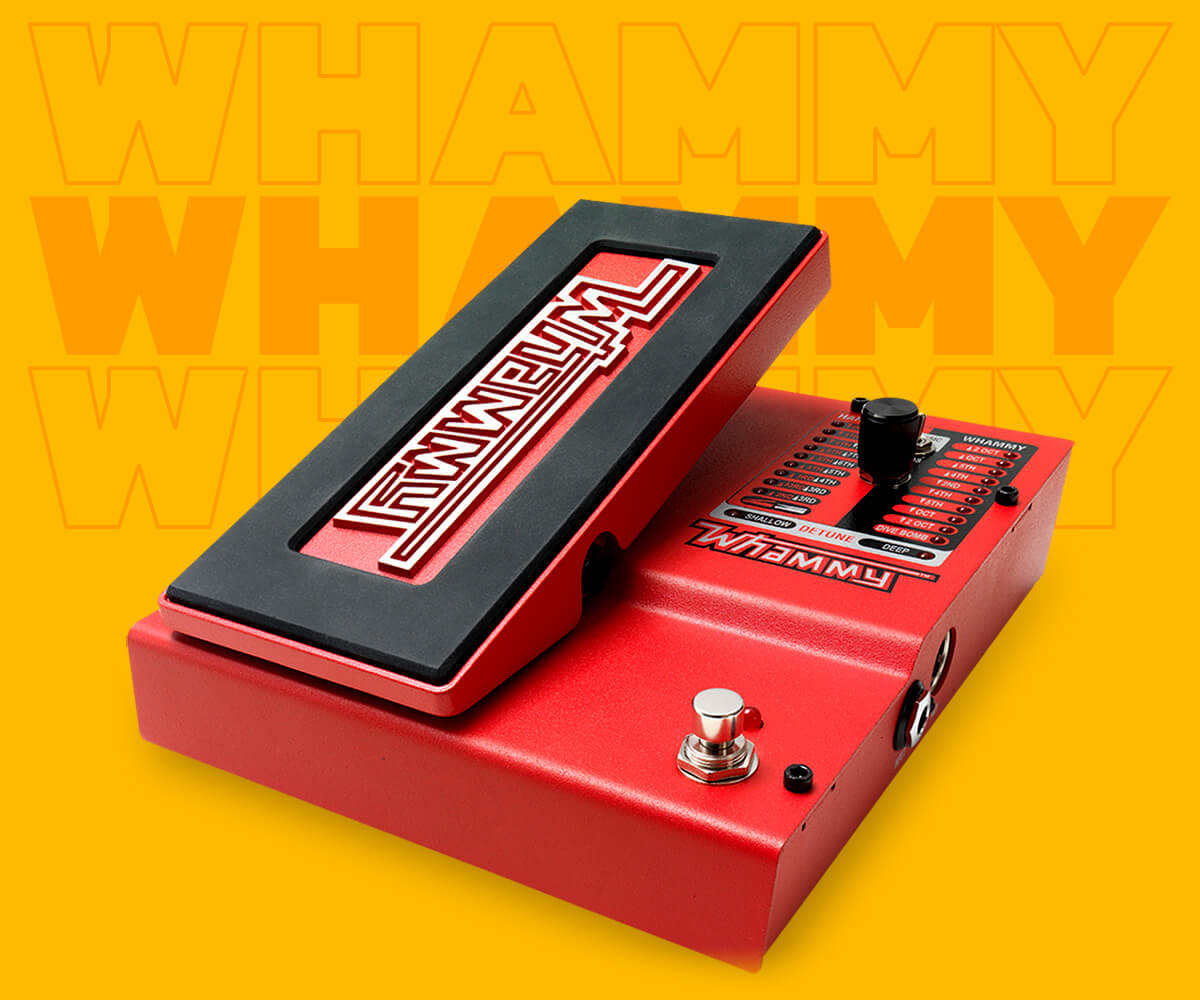This is a highly detailed photograph of a red electronic pedal device, prominently featuring the word "Whammy" in various locations and forms. The central focus is a large black and white pedal, inscribed with "Whammy" in white text. Surrounding the pedal, the device houses a black dial that adjusts settings, located at the top right corner. A small metal port and a silver bolt-like fixture are visible on the side and the bottom right corner, respectively. The background is a rich, golden-dark-yellow hue, adorned with the word "Whammy" repeated three times in a stylized yellow outline text. The repetitions are subtly varied, one being clear and another showing a shadow effect. The overall appearance suggests a sophisticated electronic equipment with intricate details, not a shoe size measuring device as initially mistaken due to the stylized logo.